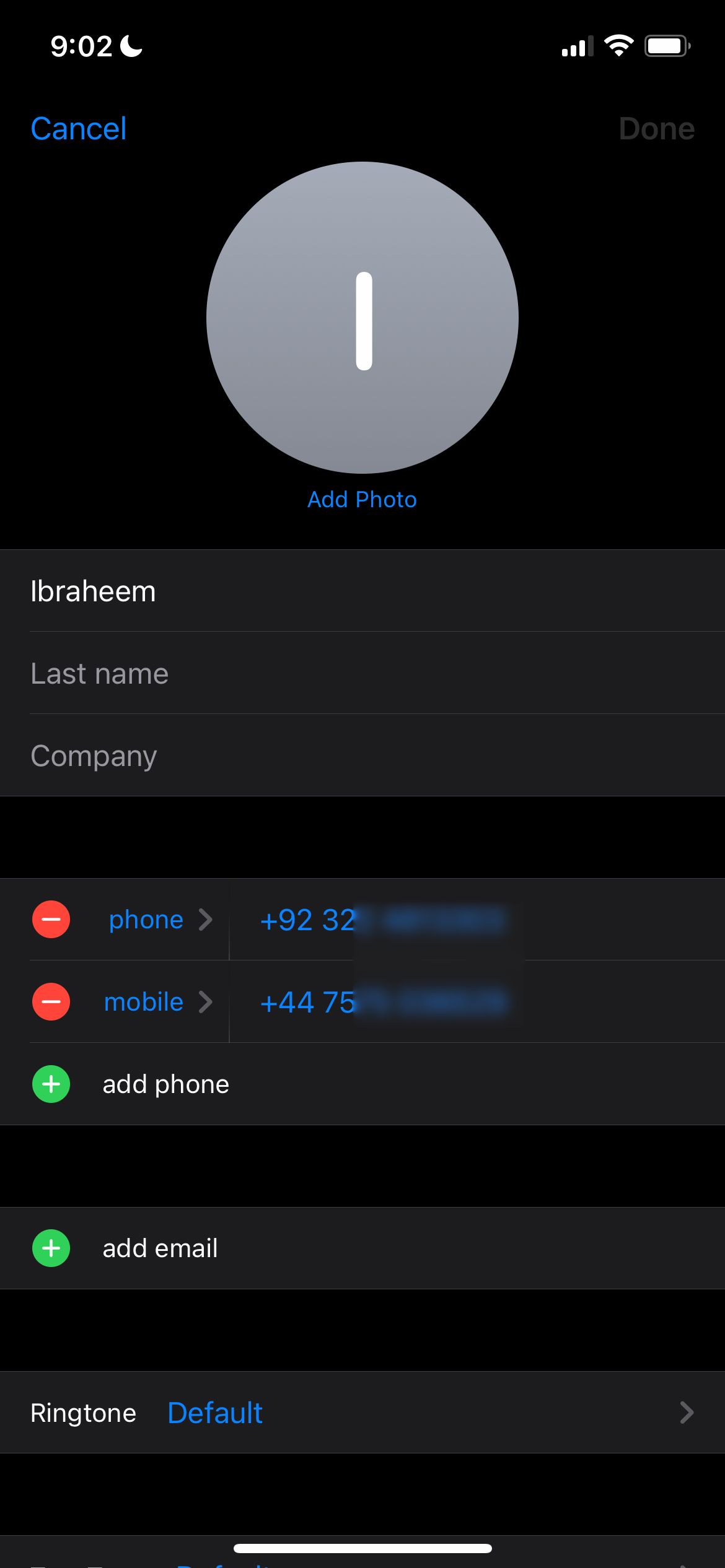The image appears to be a screenshot taken from a smartphone, displayed on a black background. At the very top left of the screen, the time is indicated as "9:02," with a moon icon to its right, suggesting it is nighttime or Do Not Disturb mode is active. On the top right, there are three signal bars, a Wi-Fi icon, and a nearly full battery icon.

Beneath the time on the left side, there is a "Cancel" button, and on the right side, a "Done" button. In the center of the screen, a large gray oval with a white square in the middle contains the text "Add Photo." This likely indicates an option to add a photo to a contact in the phone's address book.

Below this option, the name "Ibrahim" is entered, but the fields for "Last Name" and "Company" are left blank. Underneath these fields, there is a red minus sign inside an oval next to the word "Phone." The phone number displayed alongside it starts with "+9232" but is partially obscured. Similarly, another red oval with a minus sign next to the label "Mobile" shows a partially obscured number starting with "4475." 

Further down, a green plus sign in an oval labeled "Add Phone" suggests an option to add another phone number. Another green plus sign in an oval below it, labeled "Add Email," indicates an option to add an email address, though no email has been added. 

At the very bottom of the screen, the text reads "Ringtone is default for this person," suggesting no custom ringtone has been set for this contact.